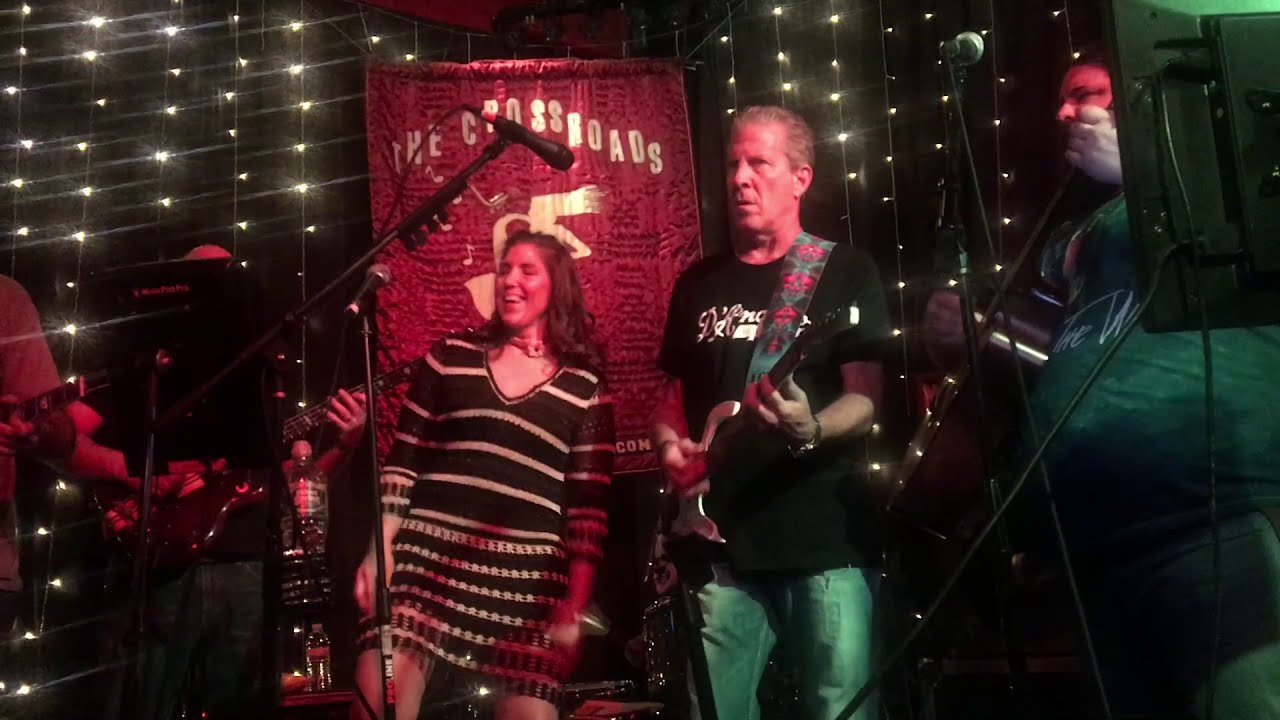In the darkened scene of this digital photograph, five performers are captured on a stage lit by numerous tiny white LED lights strung on wires against a black backdrop. Dominating the background is a prominent red banner with the golden inscription "Crossroads." At the center of the group stands a smiling woman clad in a black dress with vertical white stripes. She is positioned in front of a standing microphone, energetically singing and dancing. To her immediate right is a man playing a guitar, dressed in a black shirt with white lettering and blue jeans. Another guitar player stands to her left, also engaged in the performance. Flanking the scene, on either side of the central trio, are two more men with guitars, though their faces are partially obscured. Together, the five musicians create a vibrant and dynamic stage presence, harmonizing their melodies under the sparkling canopy of lights.